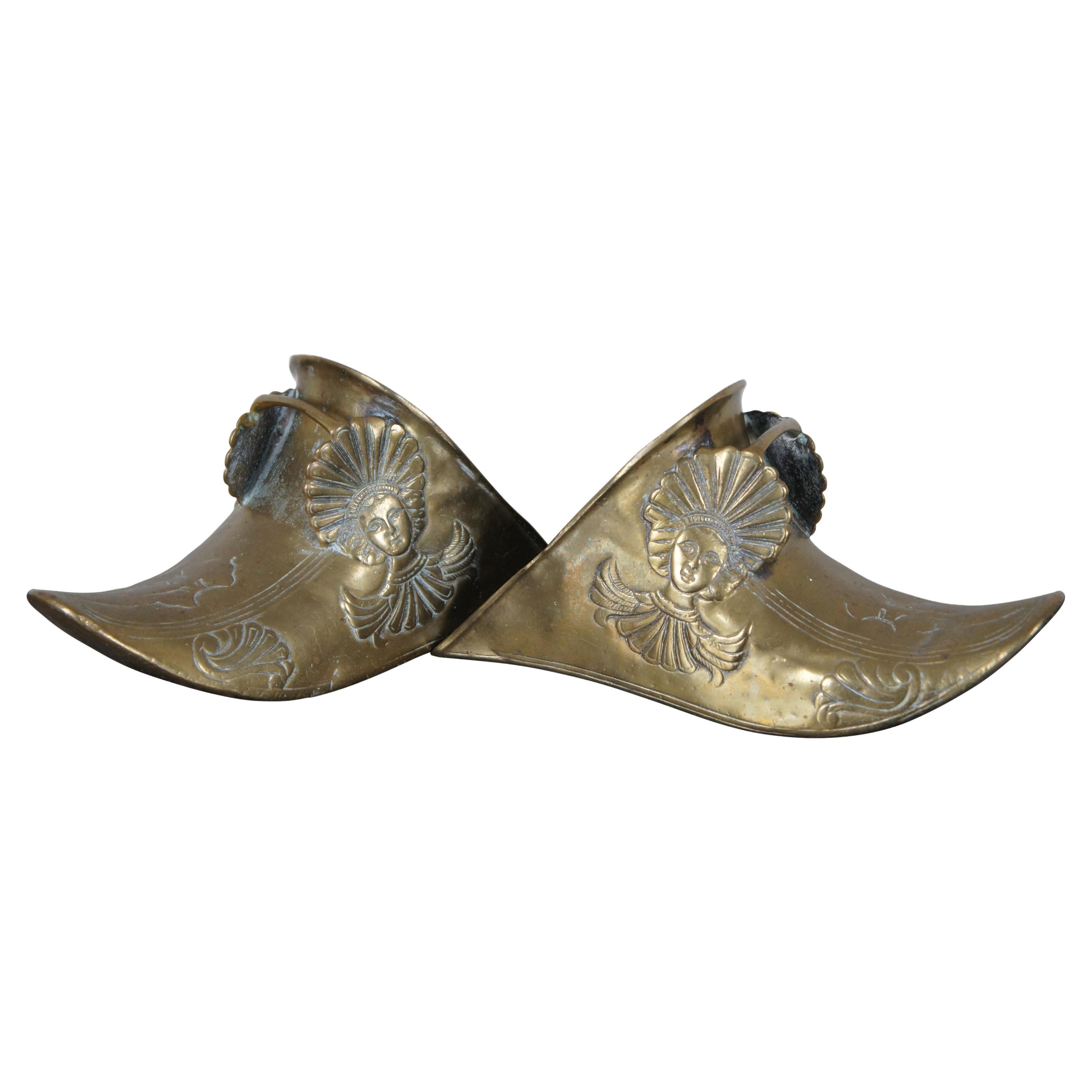The image depicts a pair of small, ornate metal objects that resemble gold or brass shoes but could also be shoulder pauldrons. Each piece has a curved, horn-like shape with a swirled tip, suggesting where toes might go if they were indeed shoes. There are intricate design elements, including a prominently featured woman in an elaborate headdress, reminiscent of ancient Cleopatra-era artistry, on each piece. These women are depicted from the neck down with their intricate clothing extending to the edges. The designs on the shoes show floral filigree patterns near the front. Both shoes display a black section on the sides, though the exact design of this part is unclear. One of the headdress designs slightly protrudes from the surface, indicating a three-dimensional aspect. The metal appears dark and not overly shiny, adding to the antique look of these possible ceremonial artifacts.